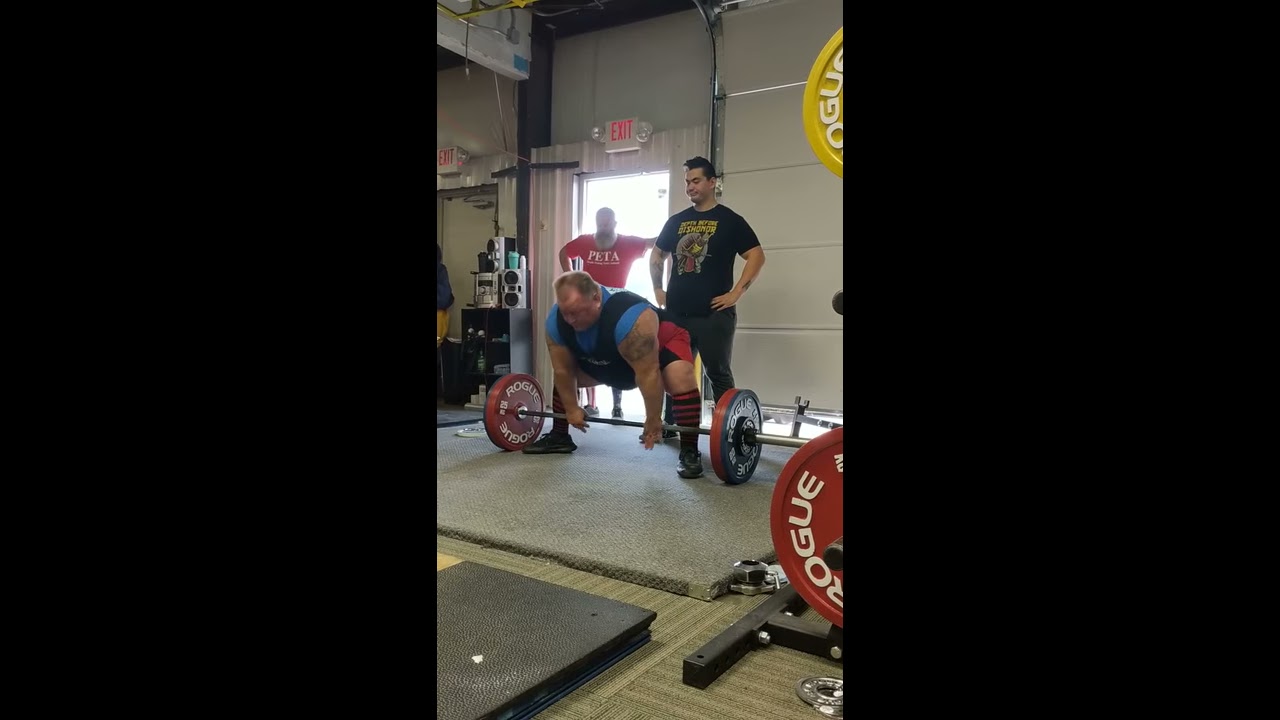In the image, a robust man, central to the scene, is poised in a deadlift position over a barbell labeled "Rogue" with red and black rings on either end. He wears a blue short-sleeved t-shirt under a red tank top, red shorts, and red and black striped socks that reach his shins. His blonde hair and a tattoo on his left arm are noticeable. The backdrop is an indoor gym, possibly a garage-style personal gym, with a concrete grey floor and various weights strewn across mats. Directly behind the man, an open doorway with an "Exit" sign is visible. Two individuals are standing behind him: on the right, a dark-haired man dressed in a black t-shirt and trousers, and on the left, a grey-bearded man in a red top with "PETA" inscribed on it. The overall ambiance is industrial with a mix of colors including black, grey, brown, red, yellow, blue, and light blue, framed by black borders on the left and right sides of the vertical cellphone-style photograph.